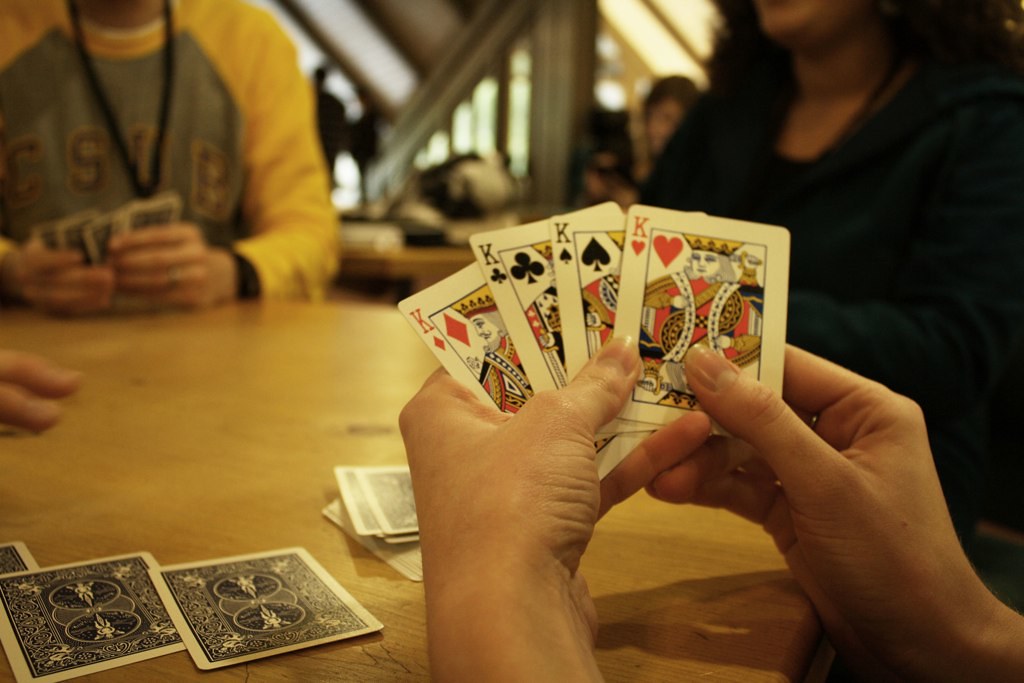In this vibrant scene captured at a table with a light blonde finish, a pair of male hands prominently holds four playing cards: the red King of Diamonds, black King of Spades, red King of Hearts, and black King of Clubs. Scattered beside him are three or four face-down cards and a small pile of additional cards bearing a distinctive blue and white pattern adorned with circular designs and a figure. Seated across from him is a man wearing a yellow long-sleeved shirt with "CSUB" inscribed on it, donning a wedding ring while he attentively holds his own cards. Adjacent to this man, a woman in a green sweater and dark hair observes the game, her hands out of sight. The atmosphere is one of quiet focus and engagement, hinting at an intense card game in progress.